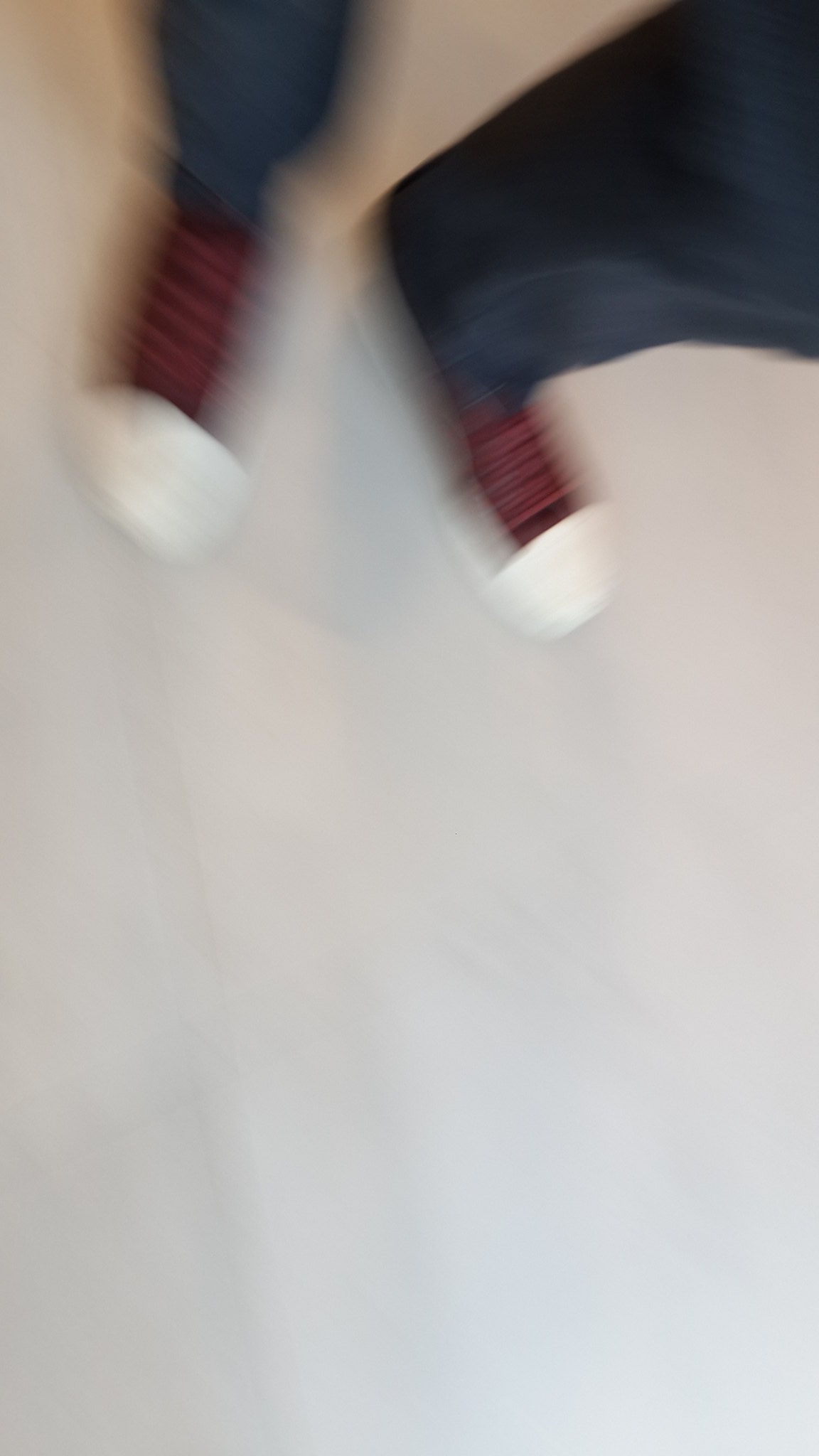The image is a highly blurred photograph primarily dominated by a light gray or white background. The top portion of the image reveals the lower half of a person's body, specifically their legs clad in blue pants. The feet are adorned with what appears to be maroon colored socks or possibly canvas sneakers, distinguished by a white toe area. The socks (or shoes) are detailed with a light-colored pattern, with the tips of the socks or the sneaker toes prominently white. The blue pant legs are only visible from the knees down, contributing to a perception that the individual is possibly in motion. The overall simplicity of the image leaves most details obscured, save for the distinct, albeit blurry, colored elements of the pants and footwear.